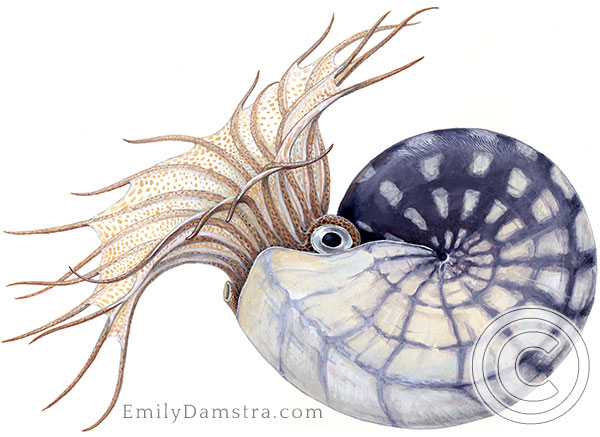This detailed illustration by Emily Damstra (emilydamstra.com) depicts a baby squid partially nestled inside a large, spiraled seashell. The shell exhibits a gradient of colors, transitioning from a creamy pearlescent hue at the outermost part to a darker, inky blue toward the center, with some descriptions noting areas of light tan or blue radiating out from the opening. Emanating from the shell's open end are the squid's many tentacles, which appear brown and are adorned with light brown spots, stretching outwards both upwards and downwards in a fanned-out manner. The squid's prominent single eye, silver with a black pupil, is also visible, adding to the lifelike depiction of the creature. In the lower right of the image, there's a floating copyright symbol serving as a watermark to protect the artwork.